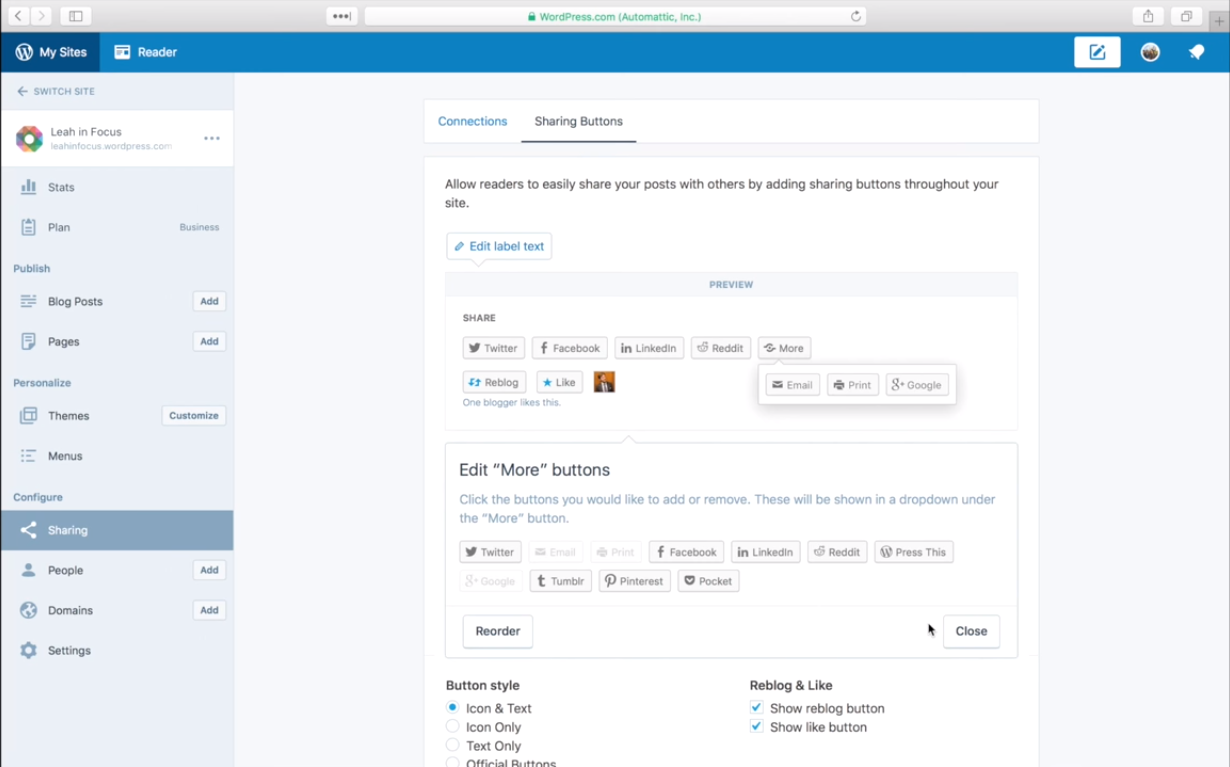This detailed caption describes the user interface of the WordPress.com dashboard, highlighting the key sections and functionalities available for blog management:

---

**User Interface Description of the WordPress.com Dashboard**

At the top left corner, the interface displays the WordPress.com logo followed by "Automattic, Inc." An arrow icon and a square icon are positioned next to it. The navigation bar is split with sections like **My Site**, paired with a blue and dark blue theme. 

Upon selecting **My Site**, a myriad of options appear including **Reader** and a notification **Bell** icon. The interface allows for site switching with a dropdown labeled **Switch Site**, followed by the site name - **focus.wordpress.com**.

In the sidebar, various color-coded menu options are listed: **Stats** to track site analytics, **Plan** to manage subscription levels, and **Business** for business-oriented tools. The **Publish** section encompasses features like **Blog Posts**, **Add Pages**, **Add Personalized Themes**, **Customize Menus**, and **Configure Sharing**.

Further down the sidebar, options such as **People**, **Domain Settings**, **Connections**, and **Sharing Buttons** are provided. Specifically, **Sharing Buttons** facilitate easy distribution of posts by adding sharing options to the site, allowing visitors to share content seamlessly.

Within the **Sharing Buttons** configuration panel, users can customize labels with an "Edit Label Text" function. Available sharing platforms include Twitter, Facebook, LinkedIn, Reddit, and more. Moreover, users can integrate additional buttons for Google, Tumblr, Pinterest, and Pocket, among others.

There are further customization options to choose the button style: **Icon + Text**, **Icon Only**, or **Text Only**. Preferences can be saved and previewed to enhance user engagement.

Overall, the user-friendly interface of the WordPress.com dashboard is designed to empower users to efficiently manage their site and optimize content sharing across multiple platforms.

---